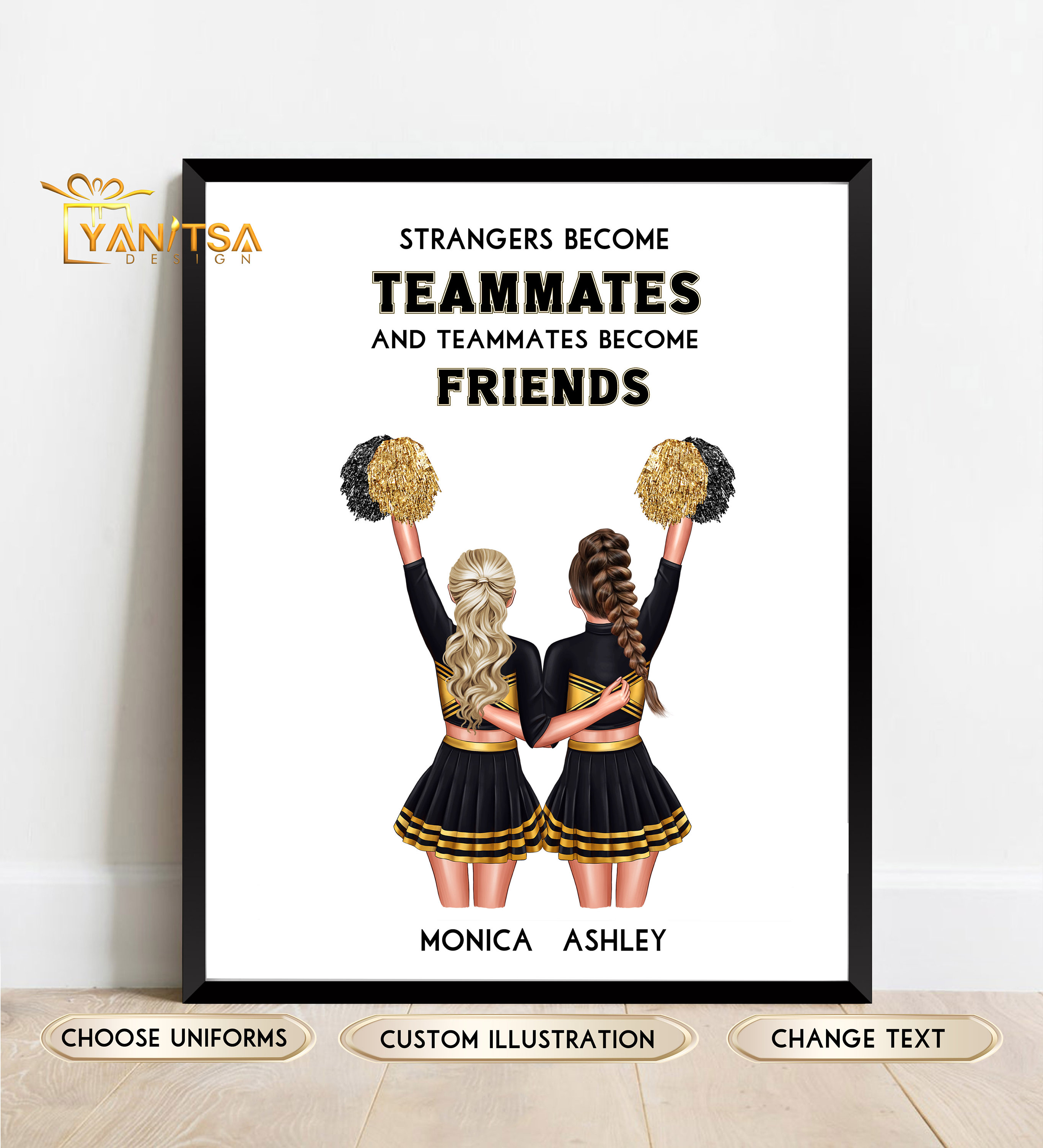The image features a cheerleading-themed artwork displayed in a black picture frame with a white background, propped against a light brown floor and a cream wall. Centered at the top of the artwork are the words "Strangers become teammates and teammates become friends" in black text, with "teammates" and "friends" emphasized in bold, uppercase letters. The illustration shows two cheerleaders standing side-by-side with their backs to the viewer, arms around each other. The cheerleader on the left has long blonde hair, while the one on the right has brown braided hair; both are dressed in matching black and gold uniforms and holding pom-poms. Beneath them, their names, "Monica" and "Ashley," are displayed. The top left of the image includes the label "YANTSA Design." At the bottom of the image, there are three interactive buttons labeled "Choose Uniforms," "Custom Illustration," and "Change Text," suggesting that this could be part of an online interface for customizing illustrations or for use in a digital game.